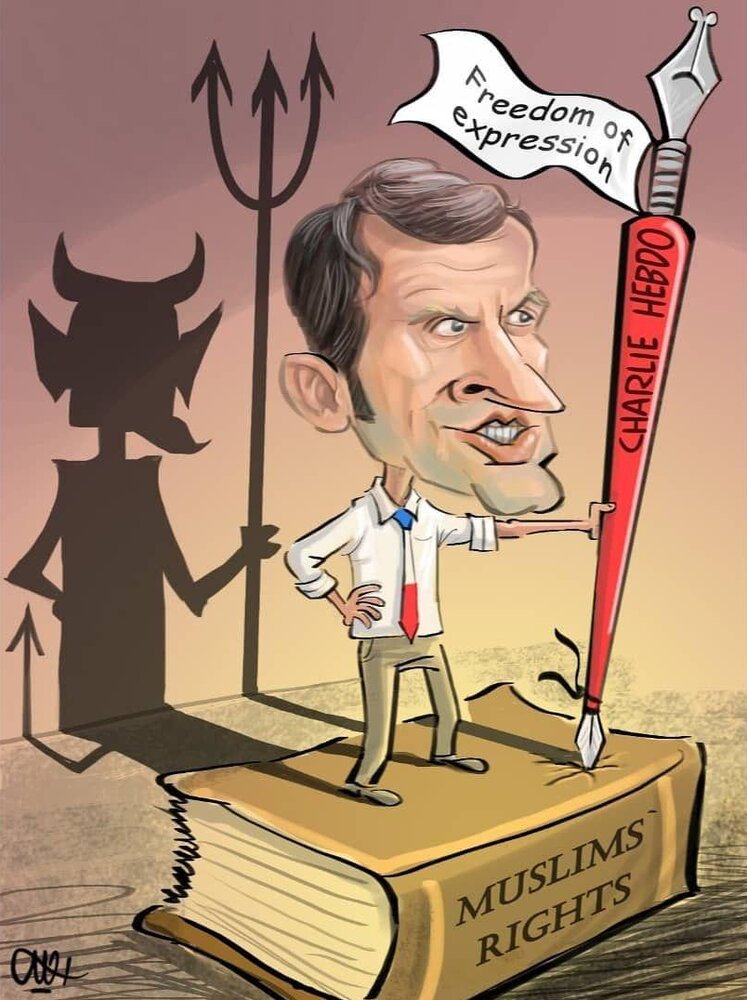This detailed cartoon image features a caricature of French President Emmanuel Macron at the center, illustrated with exaggerated facial features, including a large nose and chin. He is clad in a white shirt, red, white, and blue tie, and tan pants. Macron is depicted standing atop a large, yellow book labeled "Muslim Rights," which appears to be very thick and substantial. In his left arm, he holds an oversized ink pen inscribed with "Charlie Hebdo" and adorned with a small flag that reads "Freedom of Expression."

Behind Macron, his shadow dramatically transforms into that of the devil, complete with horns and a pitchfork, indicating a sinister undertone. This shadow is sharply cast by a light source from the right side of the image. The background transitions from a dark brown at the top, gradually fading to a lighter brown, then beige, and finally yellow near the bottom, enhancing the eerie atmosphere of the scene. The image seems to be a digitally-created cartoon, possibly published in Iran, commenting on Macron's stance and actions by depicting him as demonic.